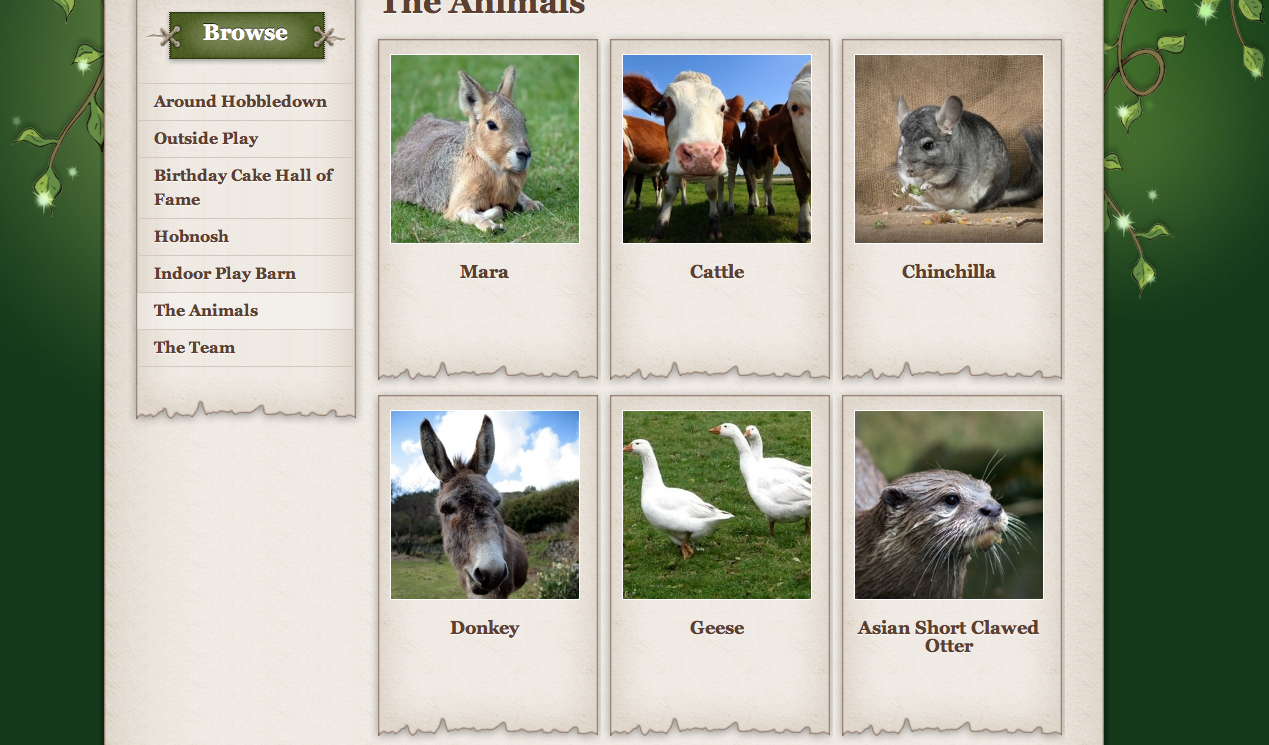This screenshot, presumably from an animal-themed webpage, presents a title prominently in the center: "The Animals." The left side of the image features a green rectangular navigation box labeled "Browse." Within this box, several page options are listed: "Around Hobbledown," "Outside Play," "Birthday Cake Hall of Fame," "Hobnosh," "Indoor Play Barn," "The Animals," and "The Team."

Dominating the central portion of the screenshot, just beneath the title, are six animal profiles, each represented by a small thumbnail image. In the top row, from left to right, are: Mara, Cattle, and Chinchilla. The second row, from left to right, features: Donkey and Asian Short-Clawed Otter. The overall design of the image showcases a background predominantly in gray or cream tones, set against a backdrop filled with various shades of green and highlighted by a plant or vine motif adorning the top corners. The menu on the left side is designed to appear like a piece of paper with a frayed bottom edge, adding a rustic touch to the webpage.